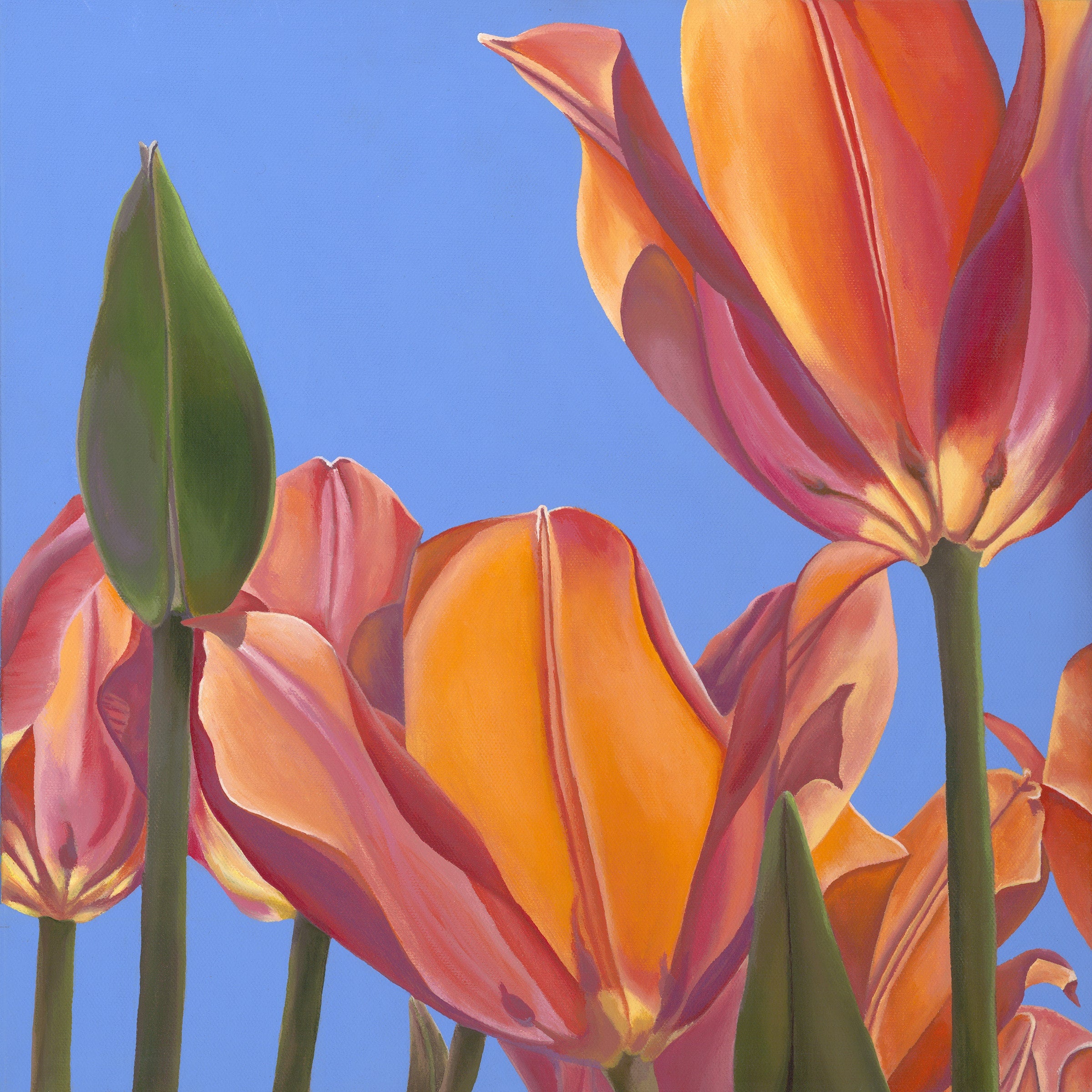This image features a striking, zoomed-in painting of a pink rose, capturing only the intricate center and its unfolding petals. The artwork, possibly created with acrylic paint or watercolor, portrays the flower in vivid detail, emphasizing the mesmerizing gradients of color. At the very core, a small dark dot is surrounded by tightly curled petals, which gradually unfurl into larger shapes as they extend outward. The hues transition from a deep reddish-pink at the center to lighter pink shades towards the edges, with hints of white where light touches the outer petals. The entire square image is dedicated solely to the rose, free of any text or background distractions, creating an intense focus on the flower's lush, swirling beauty.